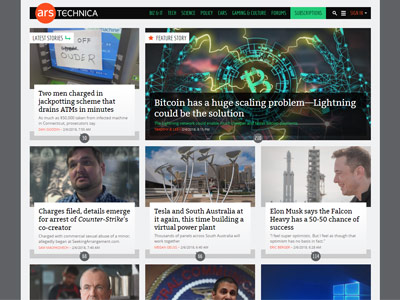This screenshot depicts the homepage of ARS Technica, identifiable by its logo in the upper left-hand corner. The layout is framed by a thin, medium gray vertical border on both sides. At the top header's right side, green headings are visible, with a green button likely labeled "Subscriptions," though the low resolution makes the smaller text hard to read.

The main content area is divided into sections, each with its own photograph. Dominating the upper right-hand section is a larger box featuring an image related to Bitcoin, characterized by a neon-colored, graphical design. This section, labeled "Feature Story," headlines with "Bitcoin has a huge scaling problem. Lightning could be the solution."

To the left, another text box highlights the article, "Two men charged in jackpotting scheme that drains ATMs in minutes." Below, three additional articles are presented in smaller squares, each with accompanying images. The headlines read: "Charges filed, details emerge for arrest of Counter-Strike's co-creator," "Tesla and South Australia added again, this time building a virtual power plant," and "Elon Musk says the Falcon Heavy has a 50-50 chance of success." Each article square is visually supported by its own relevant photograph.